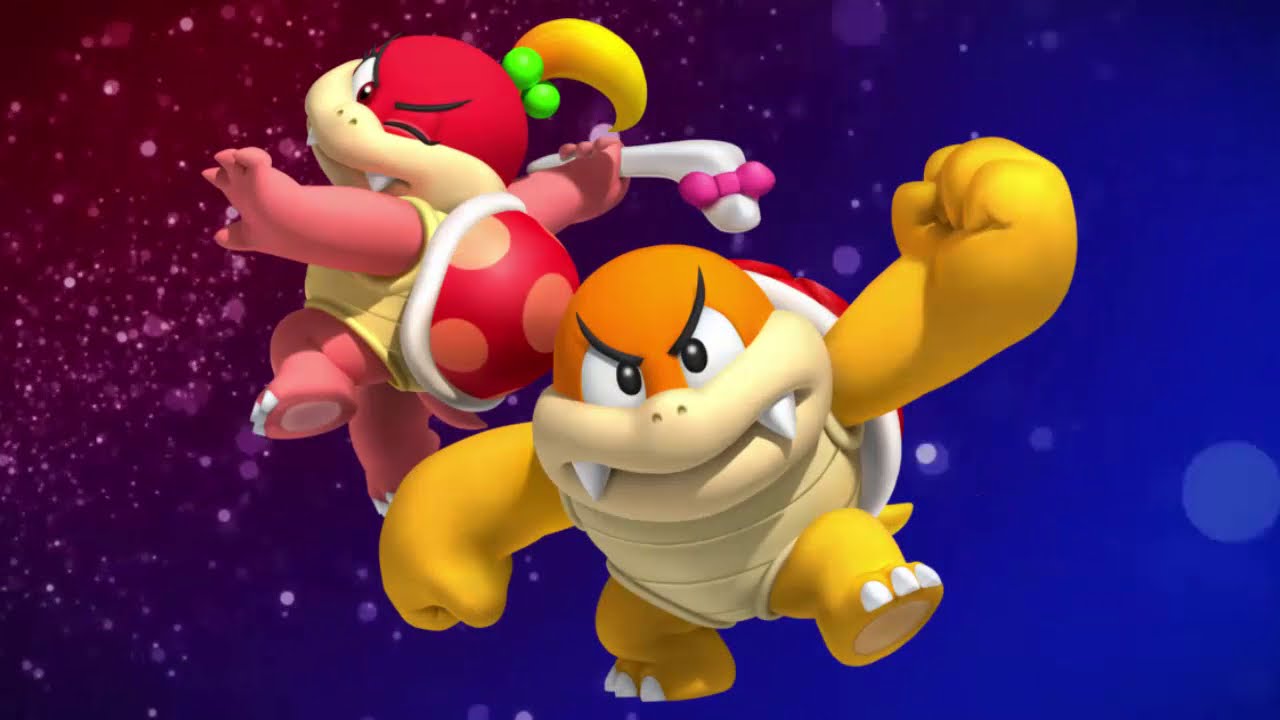In this vibrant and detailed screenshot from a Super Mario video game, we see two Koopa characters prominently positioned at the center against a vivid, split background—purple on the left and blue on the right, scattered with white dots resembling stars. The character on the right, a male Koopa, stands out with his round orange head and large white eyes. He has distinct sharp white teeth protruding from both sides of his mouth, big beige lips, yellow arms and legs, and is clad in a beige sleeveless outfit. He also carries a red shield on his back. The female Koopa on the left sports a striking red face and red limbs, contrasted by her blonde ponytail. She is holding a boomerang adorned with a bowtie, and like her male counterpart, has a red shield on her back. The image captures the essence of their cartoonish, turtle-like appearances, characteristic of the beloved Super Mario franchise.